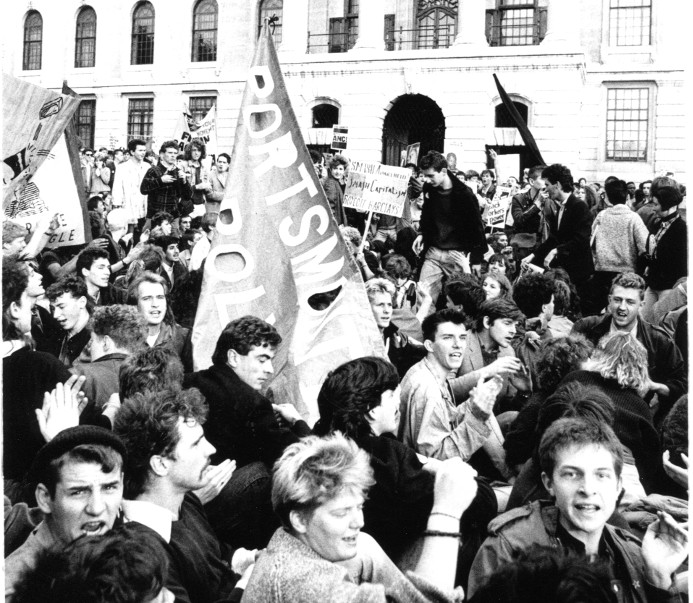The photograph depicts a dynamic black-and-white city scene filled with a large, energetic crowd. The people, whose faces occupy the entire frame, appear to be in high spirits, their mouths open as if chanting or shouting. A mix of men and women are spread out across the photo, some holding flags and signs adorned with text and art, though the exact words are unclear. The setting is a street or square in front of a white brick building with barred windows, possibly indicating an old-style construction, and suggesting the building might be institutional, like a jail. Taken during daylight, the scene's detail captures the fervor of what seems to be a protest or rally, with participants’ animated expressions and the overall sense of intense communal energy.